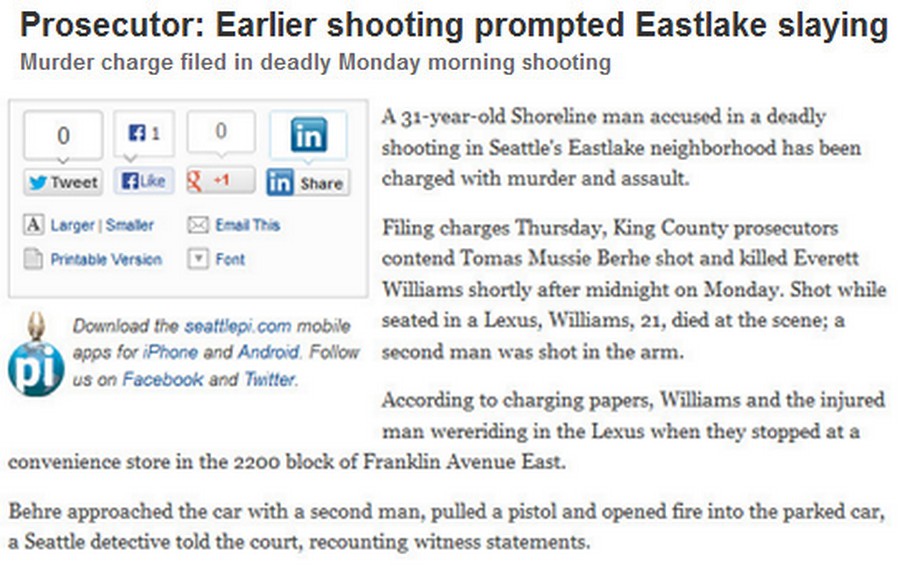An image featuring a newspaper article details a grim incident: a deadly Monday morning shooting in East Lake. The headline highlights a prosecutor's belief that a previous shooting incited this tragic event. The article, printed in Times New Roman font with black text, reports that a 31-year-old individual has been charged with murder and assault. According to the prosecutors, a woman named Everett Williams was fatally shot shortly after midnight, and a second man sustained a gunshot wound to his arm. The digital engagement for the article includes one Facebook like, zero retweets, and no other interactions from social media platforms.